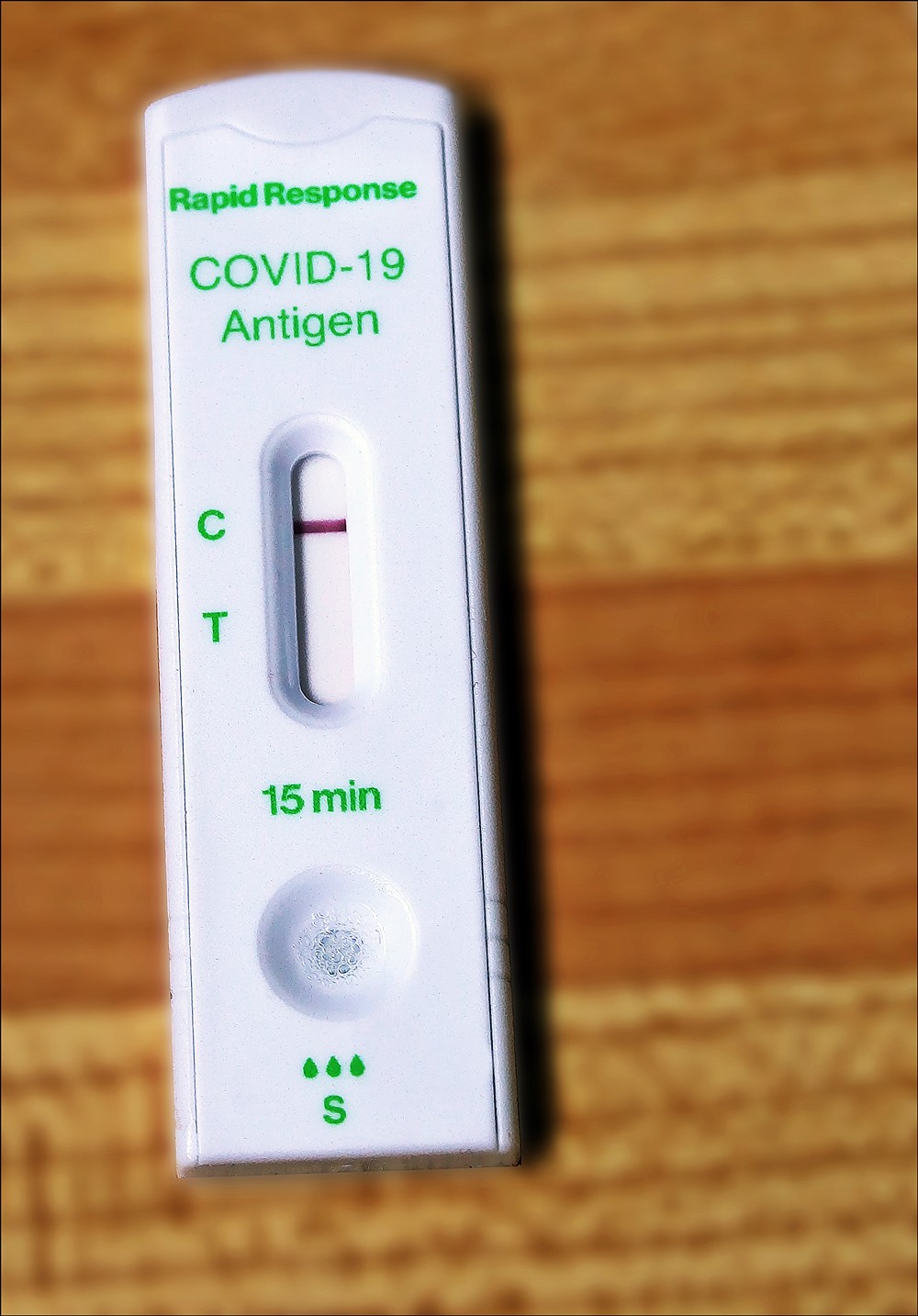This photograph captures a COVID-19 test positioned slightly off-center to the left on a wooden surface. The background appears to be composed of horizontal wooden boards, showcasing alternating shades of medium and light brown with a clearly defined grain pattern.

The test itself is a white, rectangular device with a subtle curve along the top edge. Inside this larger rectangle, a smaller rectangular section features several important details. At the top, green text reads "Rapid Response," followed by "COVID-19" repeated twice in capital letters, and then the word "Antigen."

Central to the test is an elongated pill-shaped indentation, which is recessed into the surface. Within this indentation lies a dark red horizontal line next to a green "C," with a green "T" located directly below the "C." Further down, green text indicates "15 minutes." Below this text is a white concave indentation, succeeded by three green drop symbols and the green letter "S."